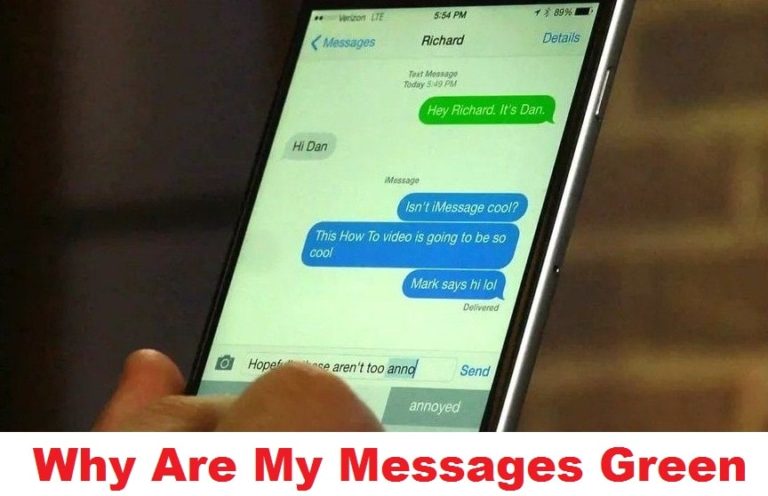The photograph features an iPhone held slightly tilted at an angle, primarily centered within the frame. The background is blurred, possibly showing brickwork. Visible at the bottom of the image, in red, sans-serif font, is the caption: "Why are my messages green?" The phone's screen displays a text conversation with someone named Richard. The status bar at the top shows "Verizon LTE" and the time is 5:49 PM. The messages begin with a green bubble saying, "Hey Richard, it's Dan." Richard's responses— "Hi Dan," "Isn't iMessage cool?", "This how-to video is going to be so cool", and "Mark says hi lol"— are contained in blue and gray bubbles. The interface suggests the phone is an iPhone, featuring iMessage, typical of Apple devices. The multi-colored text bubbles vividly highlight the central question about message color differences.